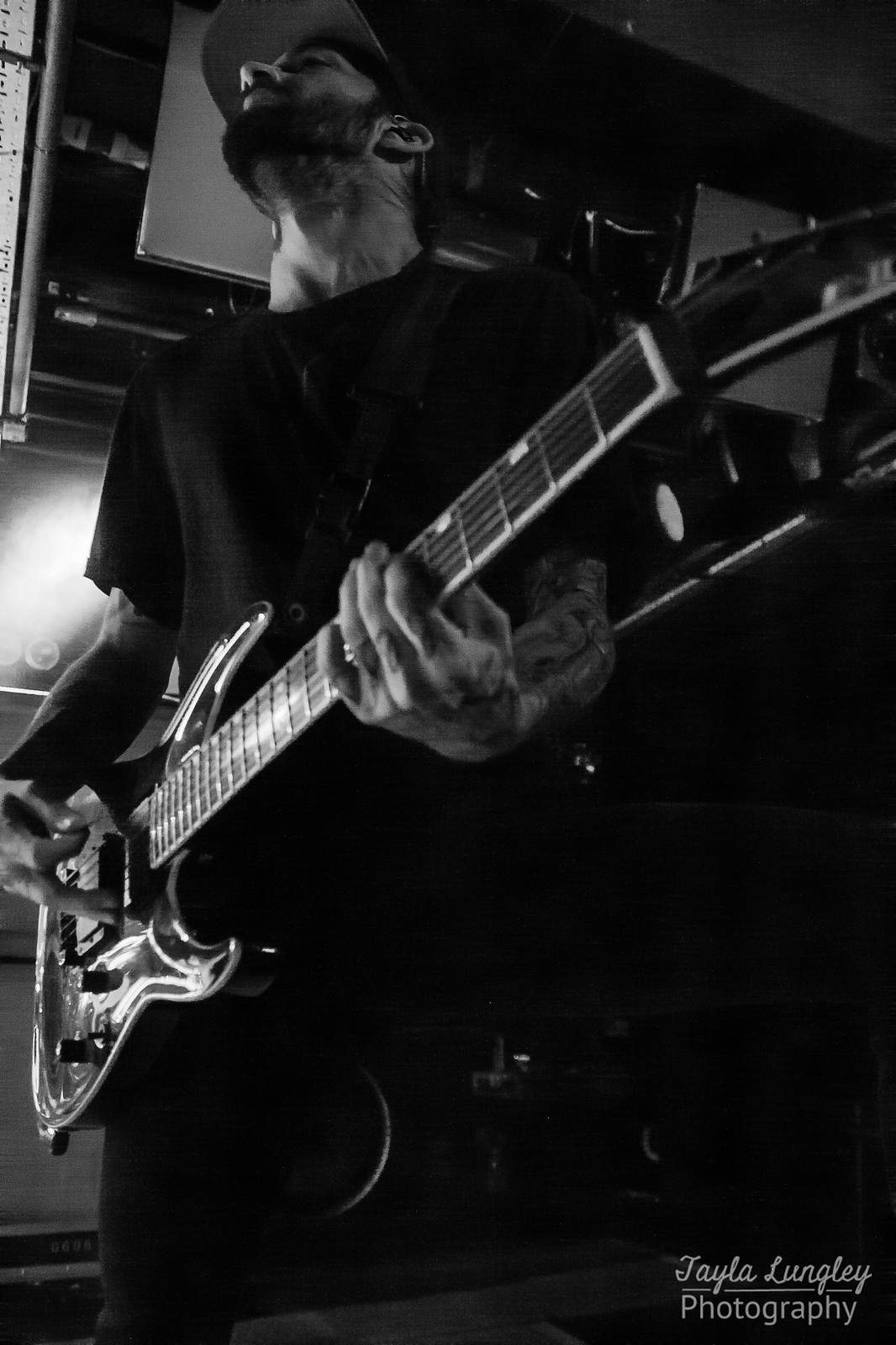In this black-and-white photograph captured by Taylor Longley Photography, a man is centered prominently in the image, holding and seemingly playing an electric guitar. He is dressed in a black t-shirt and black pants, with a cap on his head and a beard adorning his face. His head is tilted slightly upwards, with his eyes closed, suggesting he is deeply engrossed in his music. The background is dark and somewhat indistinguishable, though there are hints of an indoor setting that might resemble an auditorium or a room with shelves and lights. The overall ambiance is focused on the man and his guitar, creating a moody and introspective atmosphere.